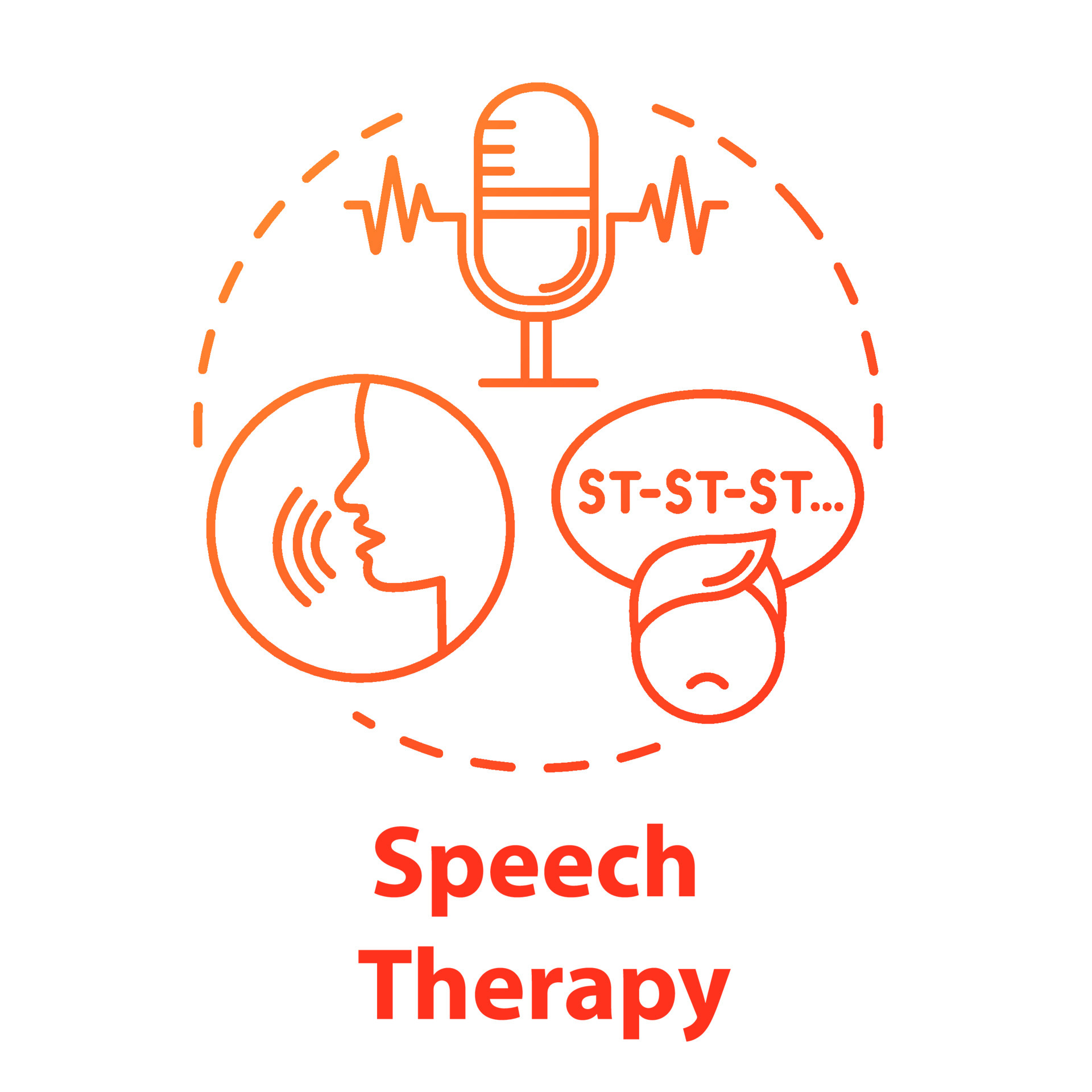The diagram titled "Speech Therapy" features an orange color scheme with a large circle made of broken lines, divided into three sections. At the top, a microphone emits dynamic sound waves. Moving clockwise, the next section shows a face with a speech bubble that reads "stuh stuh stuh," representing stuttering and signifying speech challenges. The final section depicts another face emitting radio waves from its mouth, indicating active speech. The title "Speech Therapy" is written in a gradient font that transitions from light orange at the top to red at the bottom, providing a visual cue aligned with the diagram's thematic flow. Combining these elements, the logo offers a comprehensive visual representation of speech therapy, capturing both the process and the challenges involved.